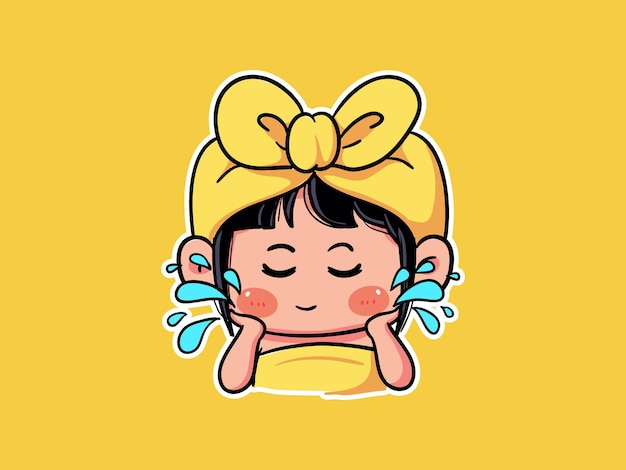This is a detailed cartoon-style illustration of a little girl against a solid mustard yellow background. The focus is from her head to just below her chest. She has a wide, squarish-round face with a cheerful expression, her eyes closed in a U-shape, and a small curved line forming a smile. Her cheeks are adorned with distinctive red blush circles. The girl has short, black hair with straight bangs peeking out under a yellow towel that's wrapped around her head and tied in a bow at the front. Wispy strands of her hair extend down on both sides of her face. She appears to be splashing water on her face, as indicated by the blue teardrop-like water droplets radiating from her cheeks. Her peach-colored skin, large ears, and indication of a yellow blouse or towel wrapped around her chest add to the lively and vibrant feel of the illustration. The entire artwork is outlined with both black and white lines, adding a distinct, bold finish to the overall graphic.